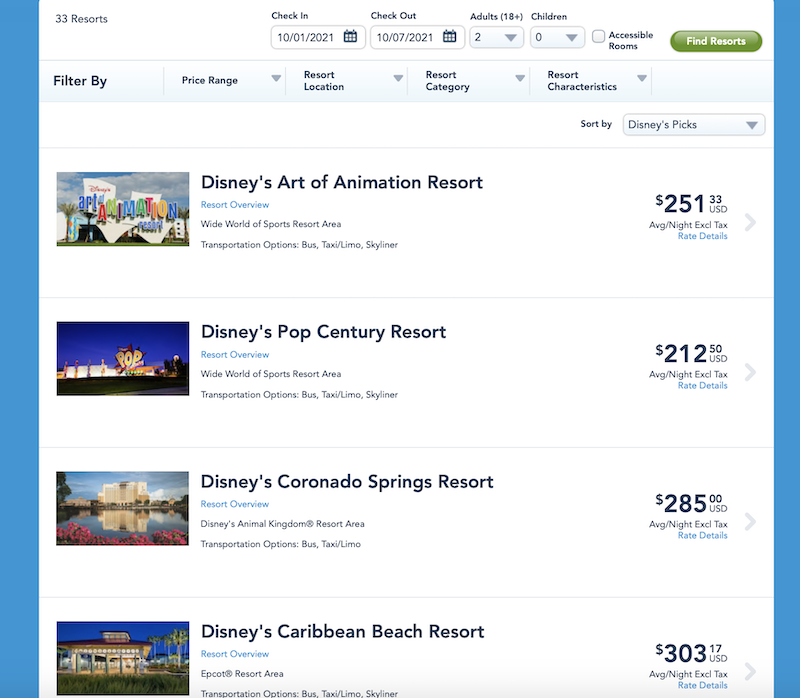This is a descriptive caption of a screenshot from a Disney vacation booking site. It outlines the available options for a stay from October 1st, 2021, to October 7th, 2021, for two adults with no children. The screenshot details four resort options out of a total of 33 listed resorts. The interface includes a green "Find Results" button, bordered by blue bars on either side. Various filters are available, such as price range, resort location, resort category, and resort characteristics, although none are selected. The results are currently sorted by 'Disney Picks'.

1. **Disney's Art of Animation Resort**:
   - **Location**: Wide World of Sports Resort Area
   - **Transportation Options**: Bus, Taxi, Limo, Skyliner
   - **Price**: $251.33 USD average per night (excluding taxes)
   - **Image Description**: A colorful sign that reads "Art of Animation"
   - **Additional Options**: Rate details, navigation arrow on the right

2. **Disney's Pop Century Resort**:
   - **Location**: Wide World of Sports Resort Area
   - **Price**: $212.50 USD average per night (excluding taxes)
   - **Image Description**: Not specified

3. **Disney's Coronado Springs Resort**:
   - **Location**: Disney's Animal Kingdom Resort Area
   - **Price**: $285.00 USD average per night (excluding taxes)
   - **Image Description**: Hotel near a placid lake

4. **Disney's Caribbean Beach Resort**:
   - **Location**: Epcot
   - **Price**: $303.17 USD average per night (excluding taxes)
   - **Image Description**: Not specified

Each resort listing includes accompanying thumbnails or photographs, headers with brief descriptive texts, and detailed pricing information positioned on the right. Additional options for rate details and navigation are available for each listing.